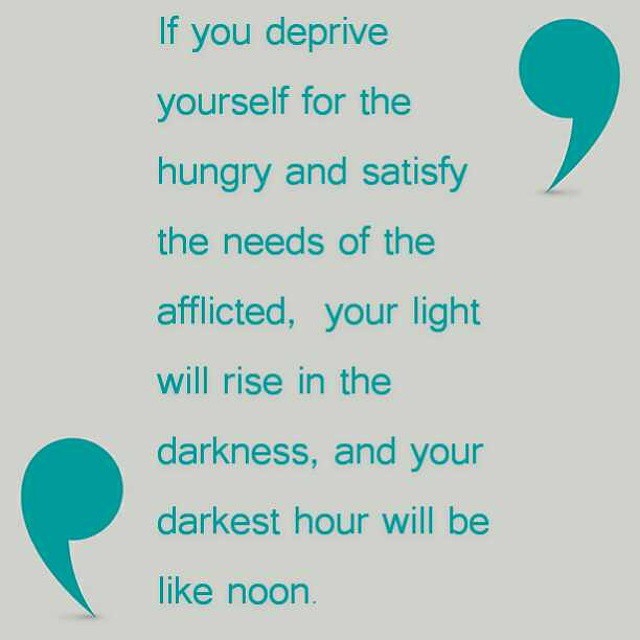The image is a square, featuring an inspirational quote that reads, "If you deprive yourself for the hungry and satisfy the needs of the afflicted, your light will rise in the darkness and your darkest hour will be like noon." The text is center-aligned, appearing in a teal color with noticeable artifacting and a slight blur around the letters. The background is a light olive-gray, contributing to the overall subdued tone of the image. Decorative oversized quotation marks in teal are positioned on the upper right and lower left corners, with the one in the lower left being upside down and accompanied by a drop shadow effect. The image is low quality with visible artifacting around the text, and there are no watermarks or additional context provided.